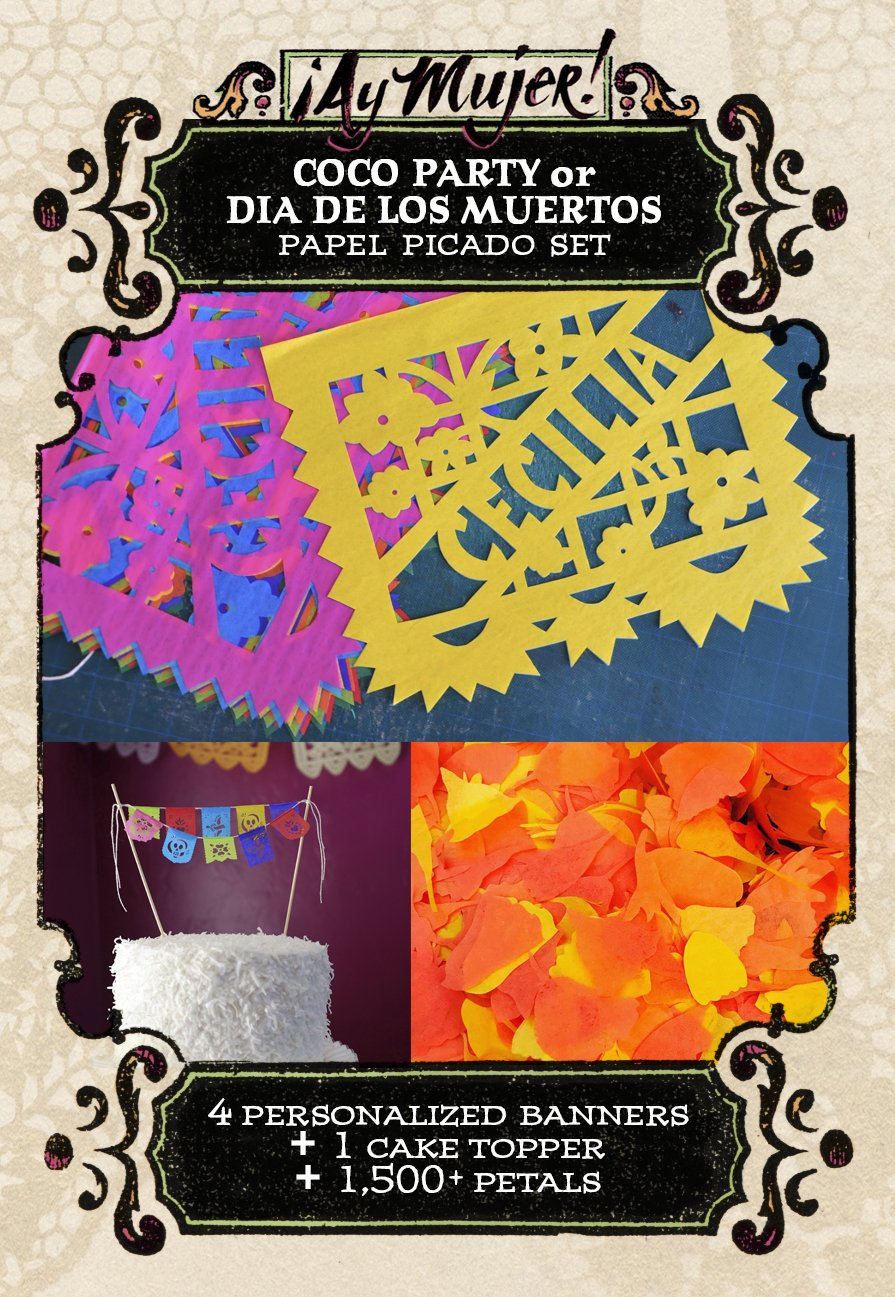This rectangular advertisement poster for a paper party set features a festive design with intricate details. The cream-colored background has a subtle honeycomb pattern at the top, which fades to a muted tone as it descends. At the top of the poster, white text reads "Hay Mujer," with a black banner underneath stating "Coco Party or Dia de los Muertos Papel Picado Set." Displayed prominently are various colorful paper decorations; a key feature being a simple cake topper banner tied to two thin skewers placed on a white cake located at the bottom left corner. Adjacent to the cake are vibrant orange and yellow flower petals made of paper. The central image includes several personalized banners with one notably reading "Cecilia." A bold black banner at the bottom of the poster announces that the set includes four personalized banners, one cake topper, and 1,500 paper petals, perfect for an elaborate celebration set.